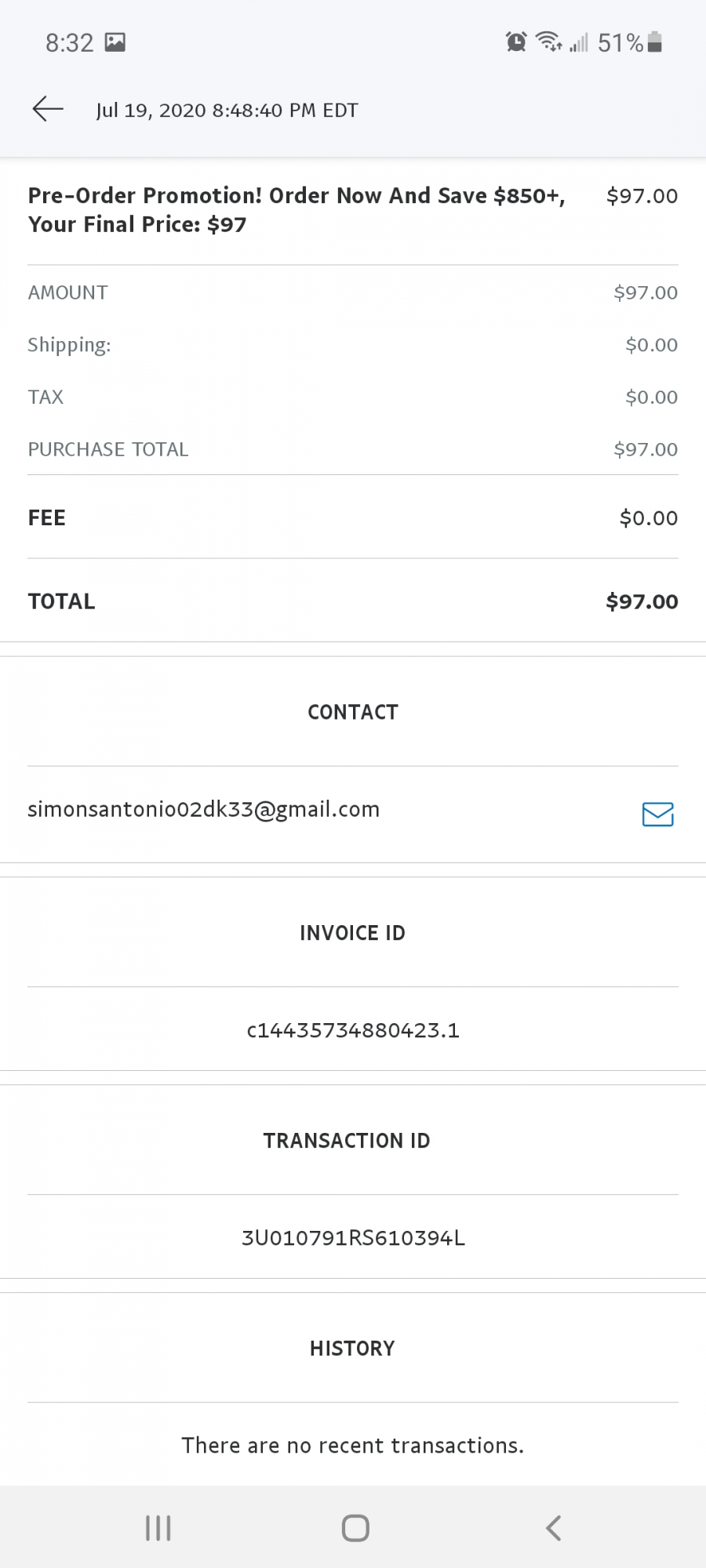This is a detailed screenshot of a smartphone screen featuring a predominantly white background with gray upper and lower borders. At the very top of the screen, the status bar displays the time "8:32" on the left side, accompanied by various icons on the right side: an alarm clock, a battery showing approximately 50% charge, and indicators for wireless and cellular connectivity.

Below the status bar, an arrow pointing left is displayed alongside the date and time: "July 19, 2020, 8:48:40 PM EDT". The main header, "Pre-Order Promotion", is bold and prominent, followed by the promotional message: "Order now and save $850 plus dollars. Your final price: $97."

Further down, a detailed breakdown of the costs is provided:

- Amount: $97.00 
- Shipping: $0.00 
- Tax: $0.00 
- Purchase total: $97.00 
- Fee: $0.00 
- Total: $97.00

Following the cost breakdown, the word "Contact" appears, succeeded by a Gmail address. Beneath this, "Invoice ID" is listed with a specific ID number, followed by "Transaction ID" with its corresponding alphanumeric code.

The subsequent section, labeled "History," indicates that "There are no recent transactions."

In the gray border at the bottom of the screen, three icons are featured: a trio of vertical lines, a square, and a small arrow pointing to the left.